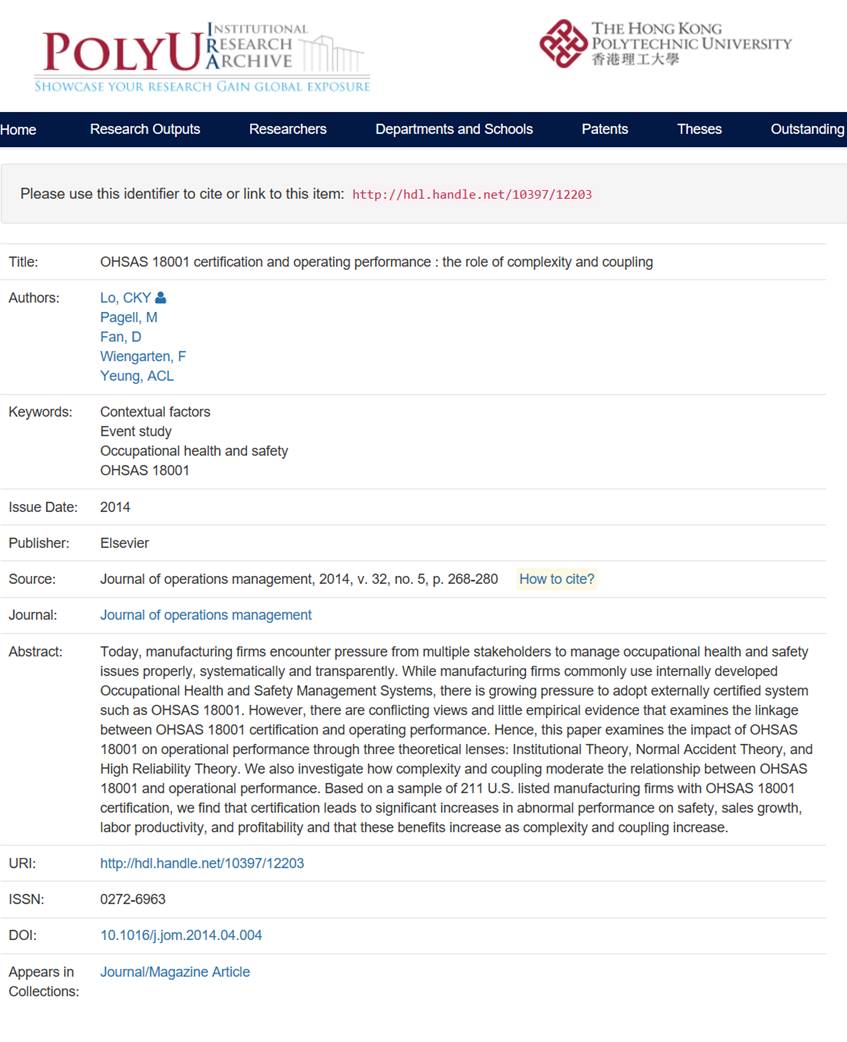A detailed caption for the image could be:

"This screenshot captures an archived article from the Hong Kong Polytechnic University website. The top of the page features a white banner displaying the PolyU logo and the text 'International Research Archive.' Below this, in blue font, it reads 'Showcase your research, gain global exposure.' On the right side of the banner is the Hong Kong Polytechnic University logo, designed to resemble a diamond with interlaced 'T' shapes, accompanied by the university’s name. Underneath the white banner is a dark blue navigation bar with white text containing buttons for 'Home,' 'Research Outputs,' 'Researchers,' 'Departments,' 'Schools,' 'Patents,' 'Theses,' and 'Outstanding.'

Beneath the navigation bar, an instruction reads: 'Please use this identifier to cite or link to this item,' followed by a URL. The title of the featured article is 'OHSAS18001 Certification in Operating Performance: The Role of Complexity in Coupling,' authored by Low CKY, Pagel M, Fon D, Wingarton F, and Young ACL. The abstract starts by noting the pressures faced by manufacturing firms from various stakeholders to manage occupational health and safety issues effectively. The issue date of the article is 2014, and it has been published by Elsevier."